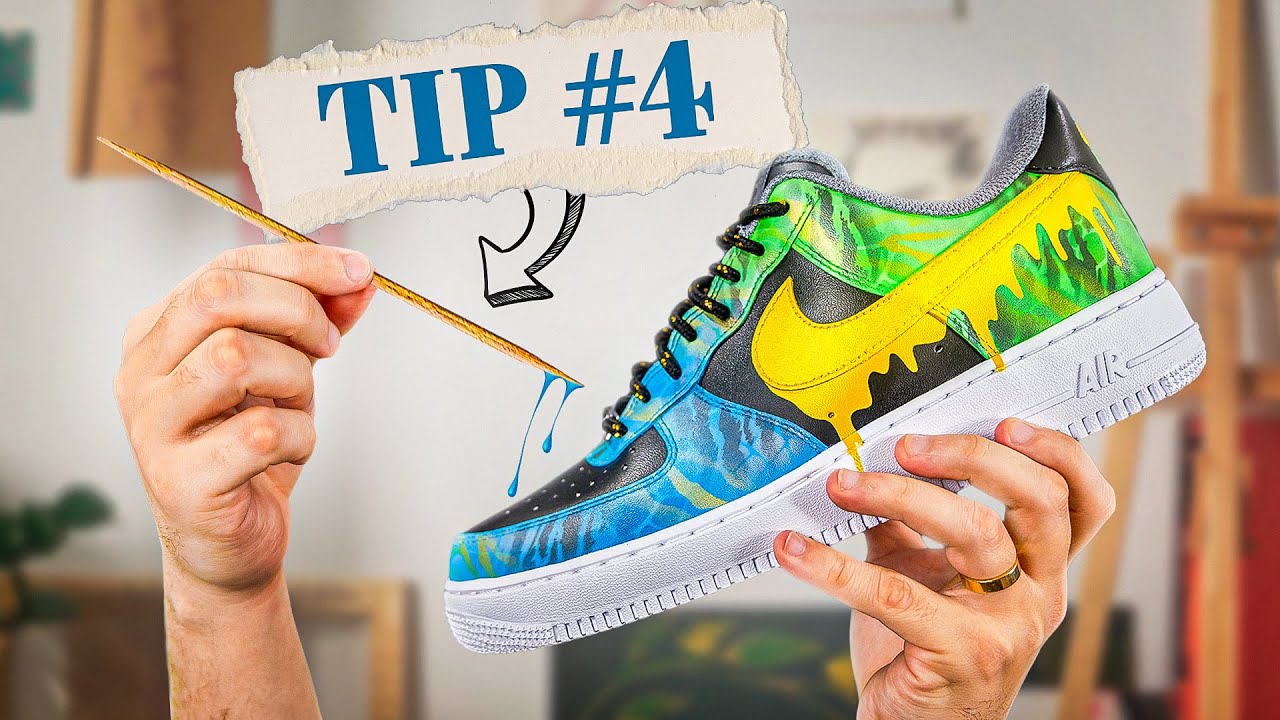The image is set against a blurred white wall decorated with framed pictures and other decor, providing a minimalist backdrop. Central to the composition are two hands, likely belonging to a Caucasian individual who is wearing a gold ring on their left hand. The left hand holds a vibrant Nike Air Force 1 sneaker, prominently featuring a multi-colored design with blue, yellow, and green paint swirls, along with a black midsection and laces. The Nike swoosh is vividly painted in yellow, with paint deliberately dripping down to create a dynamic visual effect. The shoe also has a white sole and a gray interior. Above the shoe, the right hand holds a sharp, toothpick-like stick with blue paint dripping from its tip. Large blue lettering on a tattered white background reads "tip #4," with an arrow pointing to the paint-dripping stick, suggesting a creative painting tip. The right side of the image shows a wooden frame, adding a touch of rustic charm to the overall scene.